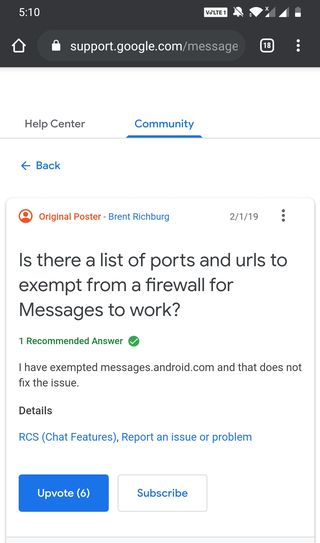The screenshot displays a section of the Google Support page dedicated to the Messages service, accessible at support.google.com/messages. The screenshot shows the top portion of a mobile device with the time displayed as 5:10, a VLTE icon, no active alarms, full Wi-Fi signal, two cellular signal bars (one low, one high), and a half-charged battery. The browser indicates that 18 tabs are currently open.

The interface is divided into two main tabs: "Help Center" on the left and "Community" on the right, with the "Community" tab highlighted in blue text. Below this, a navigation bar displays a back arrow labeled "Back," a red circular icon featuring a person symbol, and the words "Original Poster" in red text.

To the right of this icon, the name "Brent Richburg" appears in blue text, accompanied by the date "2-1-19." The main content features a query from Brent Richburg asking, "Is there a list of ports and URLs to exempt from a firewall for Messages to work?" A green checkmark denotes one recommended answer.

This answer states, "I have exempted messages.android.com and that does not fix the issue." Below this, there are additional interactive options including a blue chat link labeled "RCS chat features," a "Report an issue or problem" link, a "Subscribe" button in white with blue text, and an "Upvote" button in blue with white text showing six current upvotes. To the right of the date and name, there are three vertical dots indicating a side menu for additional options.